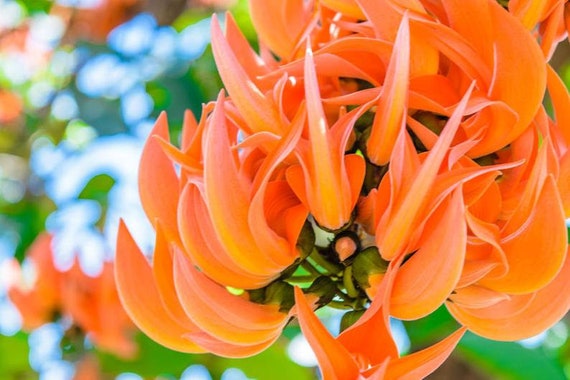This image showcases a close-up of a breathtaking tropical plant with tightly clustered, vividly colored petals that curl and fold in a ribbon-like texture. The plant's petals exhibit a striking palette of bright, vivid apricot orange, with hints of pink and coral hues, creating a high contrast against the surrounding green buds and foliage. The composition of the petals is dense and intricate, often appearing as though multiple small flowers have grouped together to form a larger, singular bloom. The background is blurred, offering glimpses of more of the same plant and patches of sky, which further accentuates the focus on the vibrant colors and delicate structure of the plant. The detailed close-up captures the organic beauty and complexity of the petals, while the softened backdrop enhances the vivid tones and textures of the main subject.